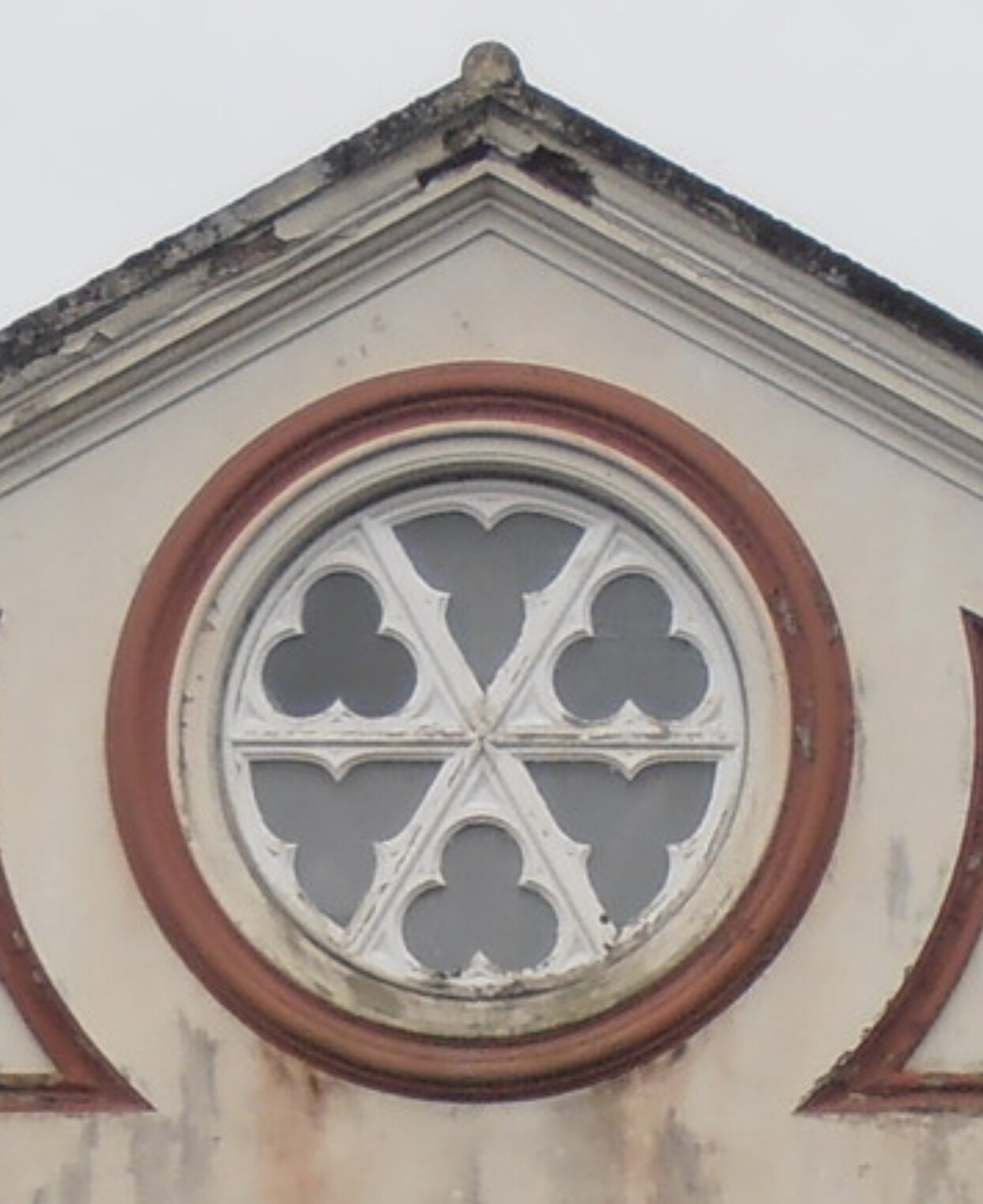The image depicts the upper exterior of a heavily weathered and aged building, centering on an intricate circular window located at the apex of a triangular roof. The roof itself is laden with dirt and blackened by time. The building’s facade is a light tan with some white trim, though the paint is peeling and mildew has accumulated, suggesting it is in dire need of cleaning. The circular window is an ornate design with multiple layers: an outer red circular frame, a cream-colored inner circle, and a white frame that contains a combination of clover and tri-flower shaped panes. There are two additional curved red lines on either side of the window, further decorating its elaborate structure. Above the building, the sky is mostly overcast, casting a grayish, white hue, confirming the photo was taken during the daytime. The mix of weathering, rust streaks, and intricate design give the building an old, yet distinctively historical look.